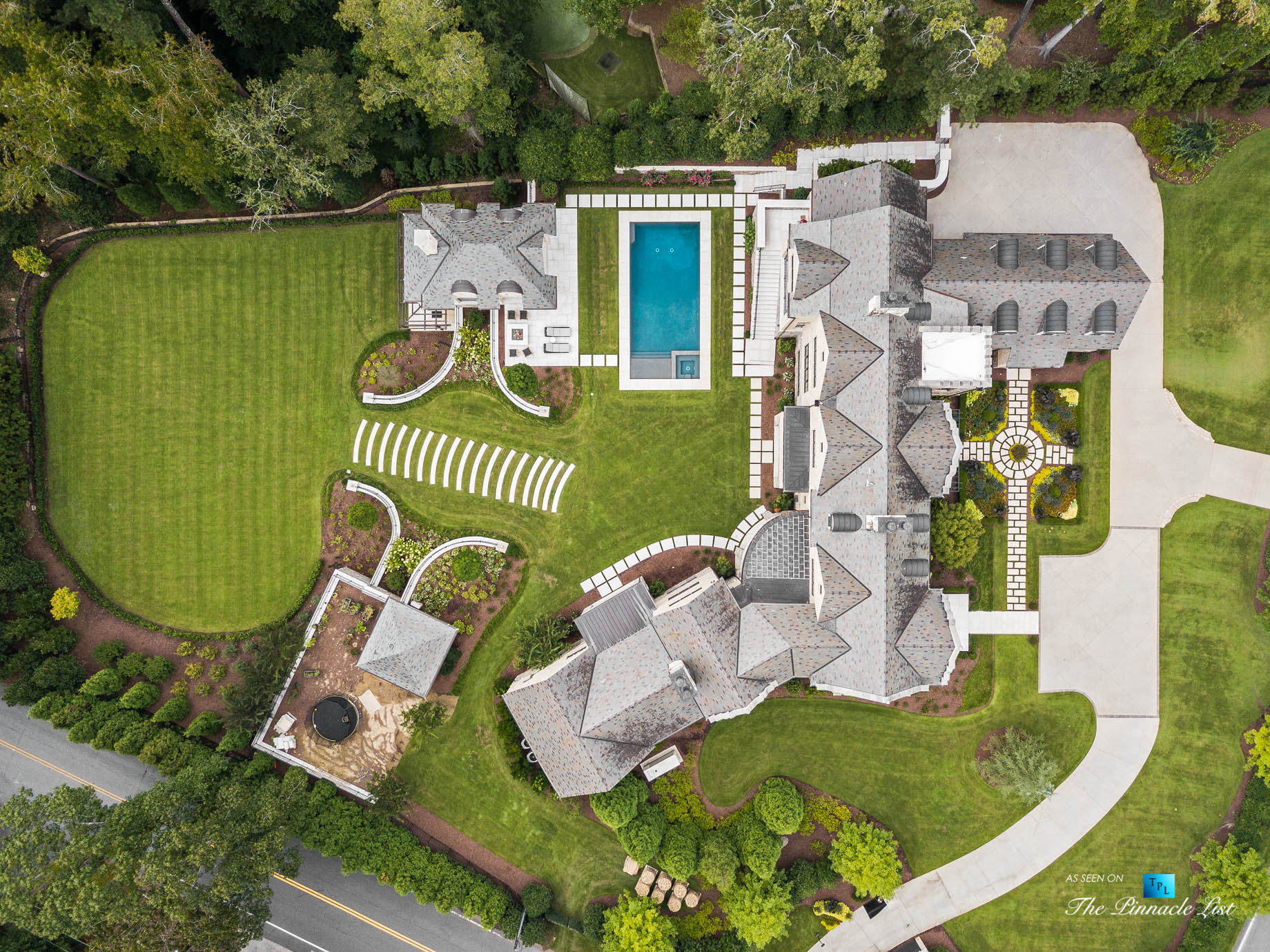The image is a highly realistic, overhead aerial photograph of an expansive mansion taken from an elevated perspective, likely by a drone, helicopter, or satellite. It captures a sprawling estate with meticulous detail, showing the top-down view of a large, L-shaped, multi-level mansion with gray roofs and white walls nestled amidst extensive green lawns. 

On the right-hand side of the image, a cross-shaped stone pathway leads to the mansion's entrance, surrounded by neatly trimmed hedges and manicured gardens. The front yard features lush green grass, while a poured gray concrete driveway is also visible. In the lower-left corner, a road runs diagonally across the corner, bordered by numerous trees that encircle the property, providing a natural boundary.

In the backyard, a crystal-clear swimming pool gleams invitingly, bordered by pathways and accompanied by a pool house or guest house. Beyond the pool, additional smaller outbuildings, which may include facilities like a jacuzzi tub, add to the estate's luxurious amenities. The backyard is vast, with more green lawns and small gardens featuring tables and chairs, highlighting a meticulously landscaped and spacious environment suitable for large events or gatherings. The upper part of the image is dominated by dense trees, further enhancing the secluded and private feel of the estate.

Notably, the image includes a small logo in the lower right corner that reads, "As seen on The Pinnacle List," accompanied by a blue square with black "TPL" lettering, indicating its feature on a prominent luxury real estate listing platform.